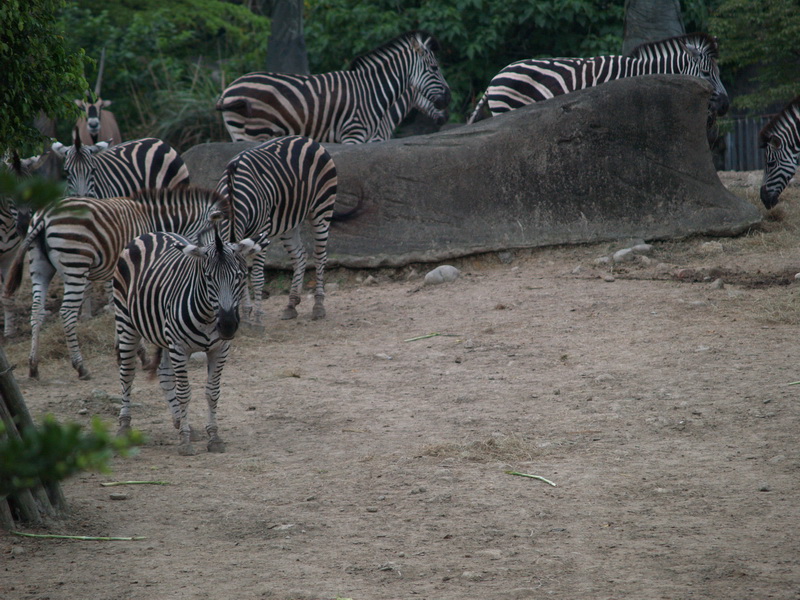This outdoor photograph, possibly taken with a telephoto lens, captures an overcast day featuring a group of zebras within a zoo or wildlife reserve. The backdrop consists of green trees and shrubbery, with an indistinct large gray object, possibly a wall or stone structure, spanning the middle. In the foreground, there is a dirt and gravel area scattered to the left. Eight black-and-white striped zebras are dispersed across the scene. Most zebras are arranged in a semicircle, with some standing idly and others walking. To the right, a distinct zebra stands in the forefront, gaze fixed directly at the camera while its tail flicks behind. Additionally, an antelope is seen faintly in the upper left, adding another layer of interest.